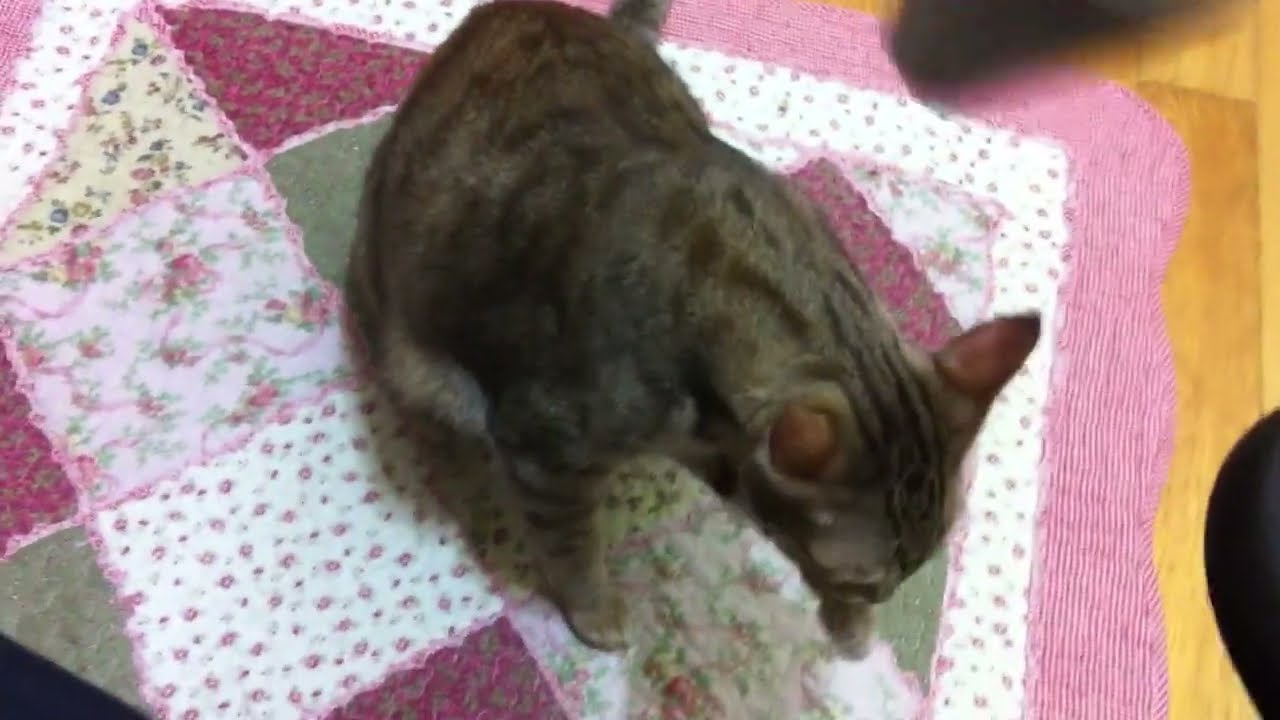In this detailed overhead photo, we see a nurturing gray and black-striped mother cat sitting on a handmade patchwork quilt. The quilt, featuring maroon and pink colors, white squares with floral patterns, and a plain pink border, rests on a light brown wooden floor inside a home. The affectionate mother cat, whose face is difficult to see as she looks downward, is nuzzling a small gray kitten. The intricate quilt also includes blue and purple accents, polka dots, and striped white and pink lines on its edges, adding a cozy, homemade feel to the setting. Some indistinguishable objects are located at the top right corner of the picture. The image captures a tender moment of warmth and maternal care between the mother cat and her kitten in a tranquil indoor environment.